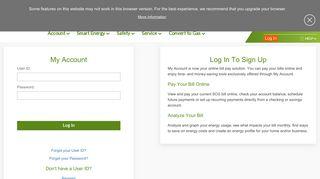The image depicts a majority white website featuring an account sign-in or sign-up page. At the very top, there is a dark grey banner with two lines of white text, which are unreadable due to the image quality. On the right side of this grey banner, there's an 'X' button to dismiss the notification. Directly below this, a white navigation bar contains a table of contents with several options written in green text, including 'Account.' To the right of this navigation bar, a green section pops out with an orange 'Login' button and a language selection feature marked by a white button. 

The main content beneath this header section is divided into two parts: on the left, a white box set against a beige background is dedicated to account sign-in. It features fields for 'User ID' and 'Password,' accompanied by a green 'Login' button. Below these fields are links for 'Forgot User ID,' 'Forgot Password,' and a prompt saying 'Don't have a User ID?' 

On the right side of the page, there's information about the sign-up process, with a header encouraging users to log in or sign up. This section highlights the benefits of online account management, such as paying bills and analyzing billing information.